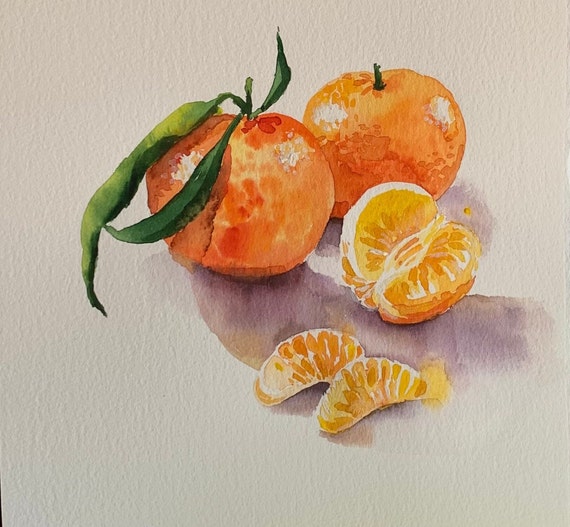This image is a detailed, square-format watercolor painting of vibrant citrus fruits set against a light tan background. The main subjects are two full-size, golden-orange fruits with darker red lowlights. The fruit on the left features a short stem with three elongated, dark green leaves, while the one on the right is adorned with just a short stem. Positioned slightly in front of these whole fruits is a half-section of the fruit, revealing its bright orange interior and white highlights, turned sideways to the viewer. On the table, in front of this half-section, are two smaller, separated slices of the fruit. The composition captures the reflection of light on the fruits, creating distinct white highlights and shadows, with the light appearing to come from the left. The overall color palette and shadows suggest a delicate balance of light and texture, presenting a lifelike and radiant depiction of the citrus fruits in this artist's rendering.